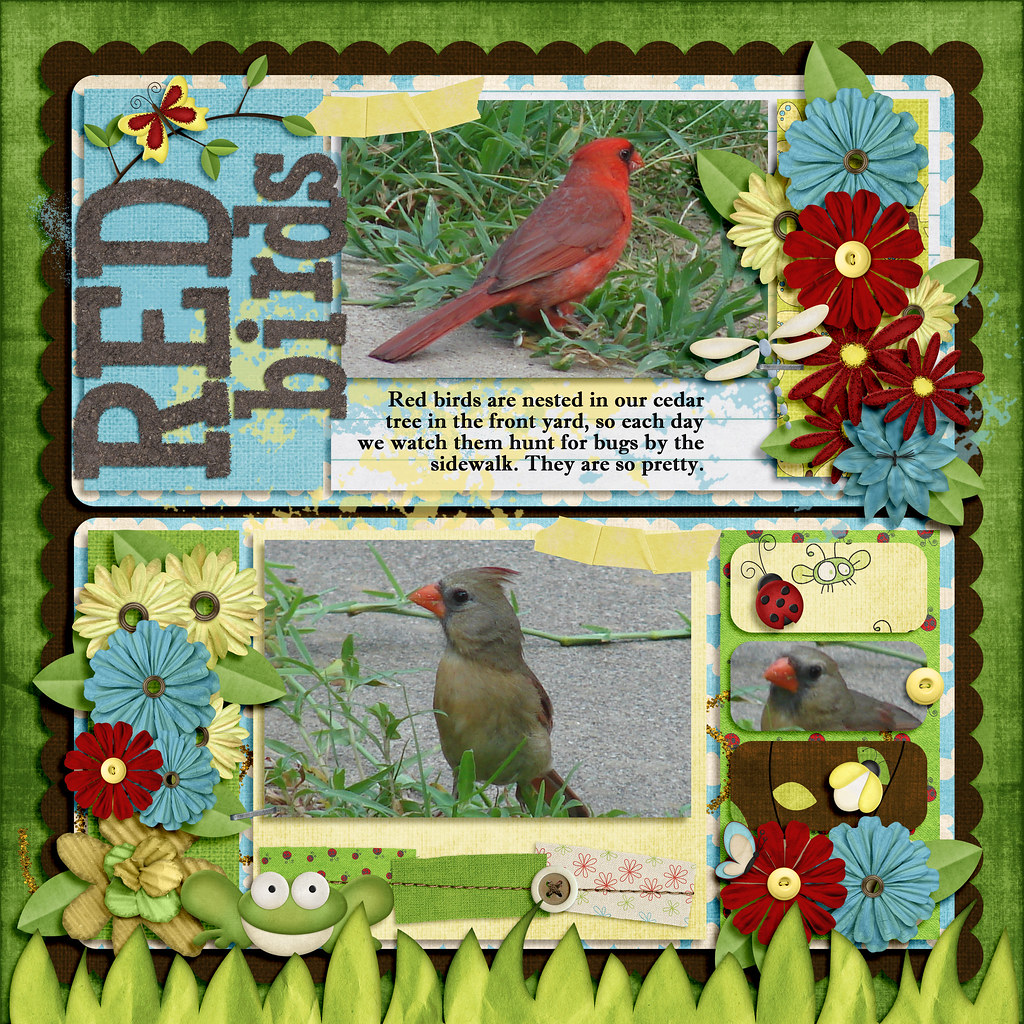The image showcases an artistic nature-themed scrapbook collage set against a textured green background, complete with digitally produced or cut-out grass at the bottom. Central to the image is a brown-framed section divided into two parts. The top portion features the words "Red Birds" written vertically on the left, accompanied by a real-life image of a red bird against a backdrop of green, black, red, and yellow colors. Below, a caption in black text reads: "Red birds are nested in our cedar tree in the front yard, so each day we watch them hunt for bugs by the sidewalk. They are so pretty." The bottom section displays an image of a gray bird, with another similar picture of the same gray bird positioned to the right.

The entire setting is designed to resemble an art project, using materials like felt to create cutesy elements such as flowers, butterflies, trees, frogs, ladybugs, and flies. The style suggests a scrapbook aesthetic, highlighting the beauty of nature through whimsical and colorful drawings, along with descriptive passages about the birds.